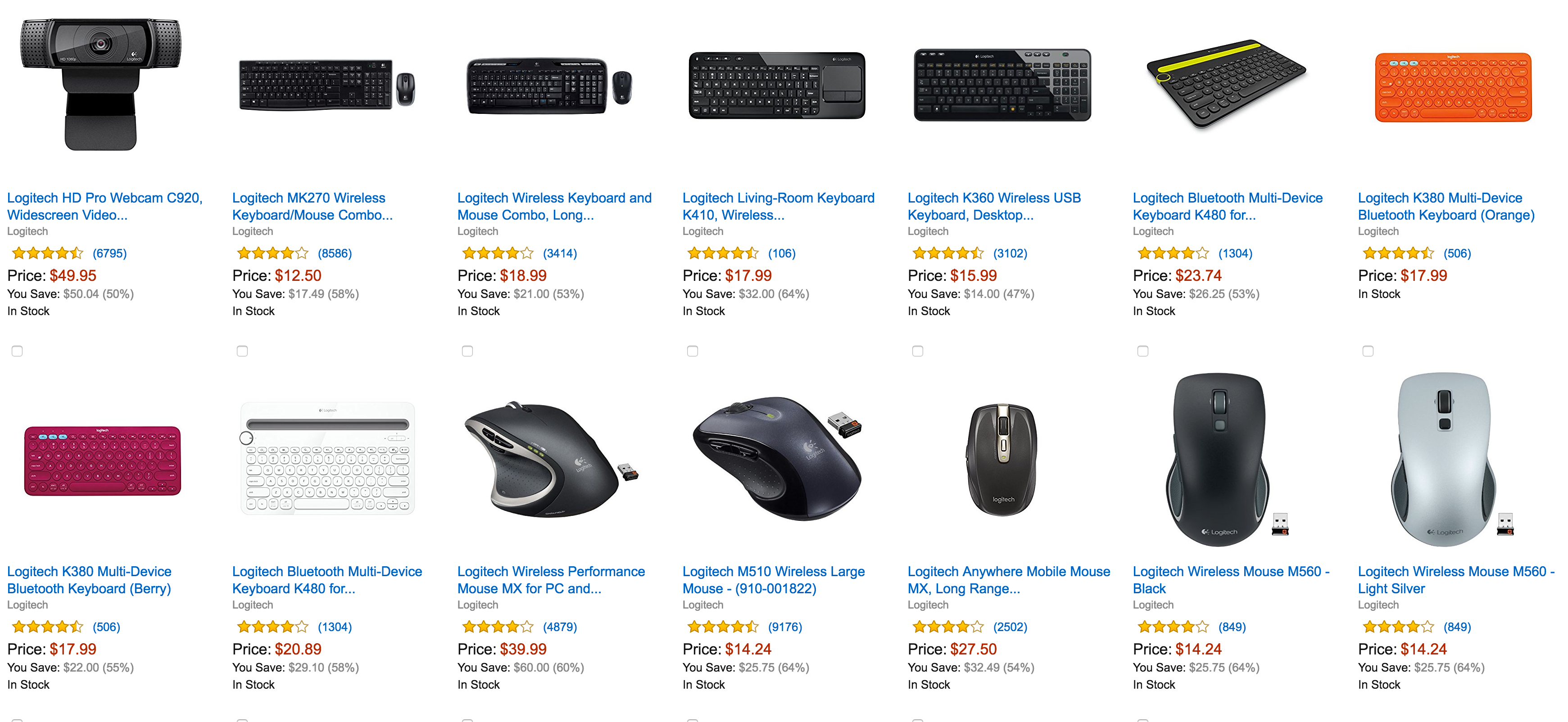### Detailed Descriptive Caption

This image is a screenshot of an Amazon page displaying various computer components. The layout consists of two rows, each with seven thumbnail images of different products. Starting from the top row, the items are as follows:

1. **Logitech HD Pro Webcam** priced at **$39.20** with a rating of **4.5 stars**.
2. **Logitech MK270 Wireless Keyboard Mouse Combo** priced at **$49.95** with a rating of **4 stars**.
3. **Logitech Wireless Keyboard and Mouse Combo** priced at **$12.50** with a rating of **4 stars**.
4. **Logitech Living Room Keyboard K410 Wireless** priced at **$18.99** with a rating of **4.5 stars**.
5. **Logitech K360 Wireless USB Keyboard** priced at **$15.99** with a rating of **4.5 stars**.
6. **Logitech Bluetooth Multi-Device Keyboard** priced at **$23.74** with a rating of **4 stars**.
7. An **orange Logitech keyboard**, possibly the Logitech K380, priced at **$17.99** with a rating of **4.5 stars**.

In the second row:

1. **Purple keyboard**
2. **White keyboard**
3. Five different types of **mice**.

Each product in the image has a brief description below it, along with its price and rating. The text appears quite small and difficult to read, especially in the bottom row, which contains the additional keyboards and mice.